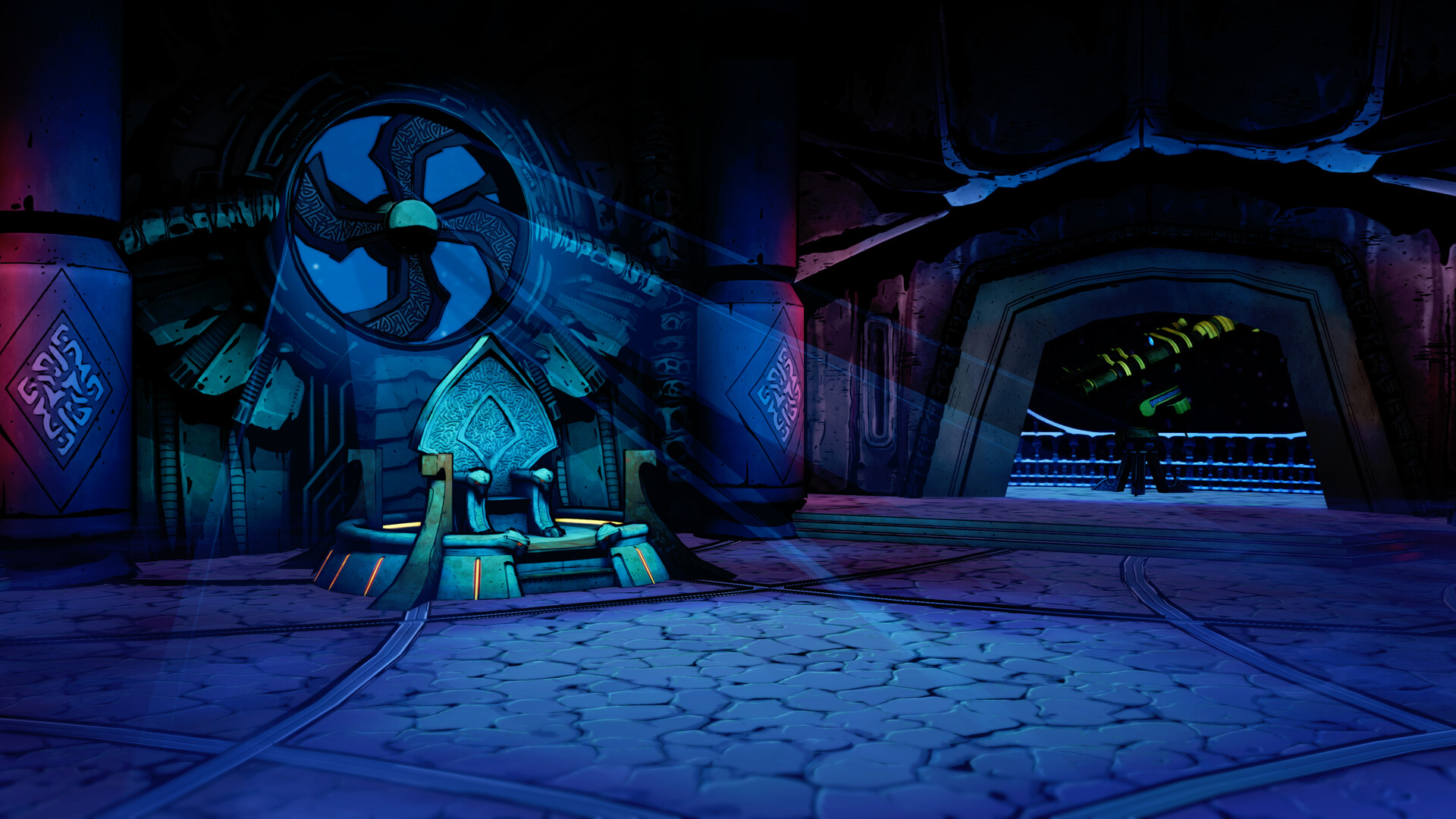The image depicts a cartoon-like, visually stylized room that suggests a throne room or possibly an area within a spaceship, characterized by a throne-like blue seat made of stone or metal. Moonlight seeps through a window designed like a fan with four blades, casting intricate shadows and streams of light onto the throne and the flat stone floor. The walls appear chiseled, featuring detailed graphic designs, giving the room a cave-like or rock-hewn ambiance. To the right, an opening leads to a balcony where a telescope (or possibly a gun) is positioned, accessible through the doorway. The overall color palette includes blues, purples, and blacks, enriching the scene with a mysterious, almost ethereal quality.